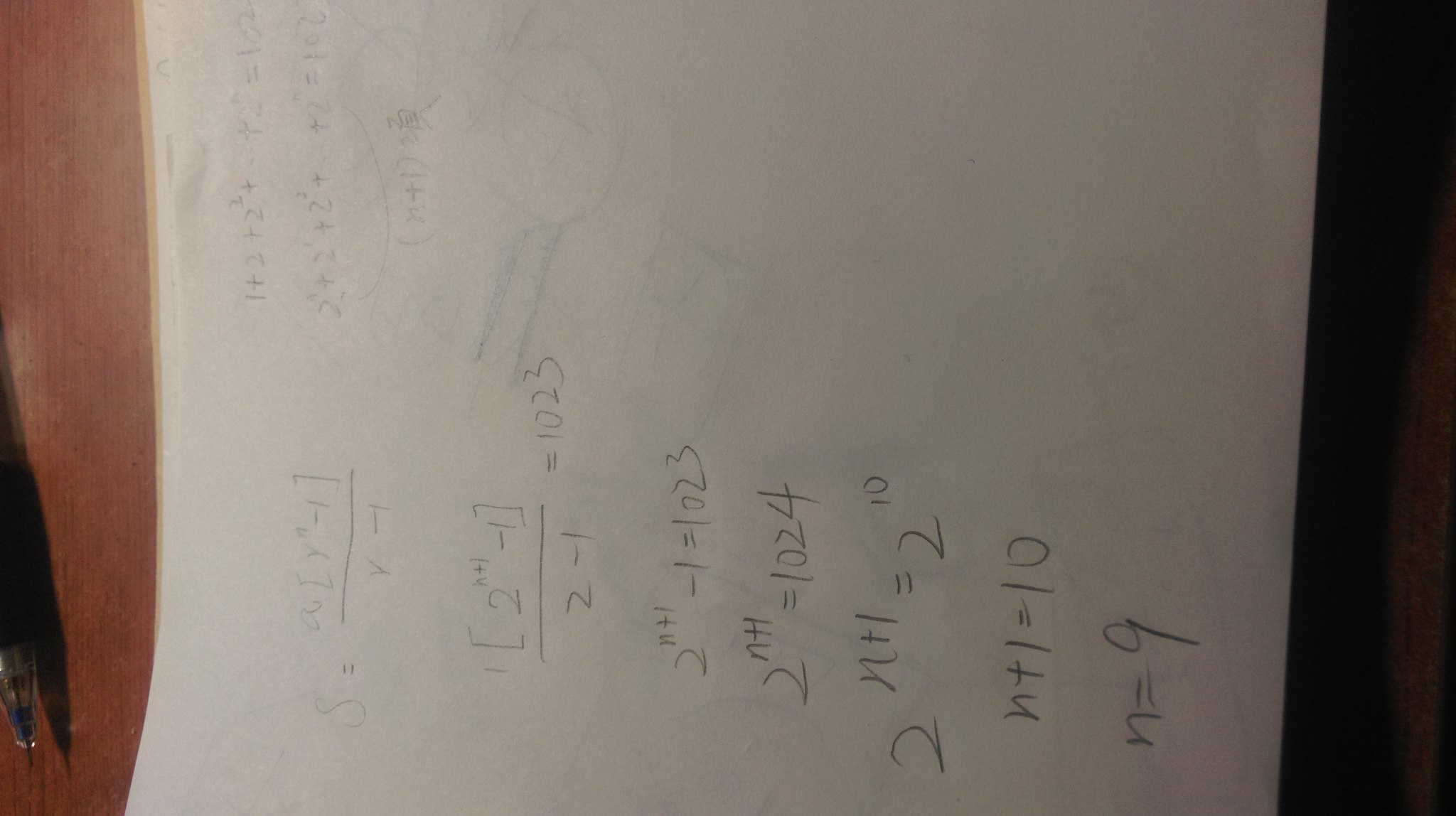This detailed top-down photograph captures a piece of paper positioned horizontally on a wooden table, showcasing a series of step-by-step mathematical equations. Just above the paper, a mechanical pencil is resting on the table, suggesting recent or ongoing work. The first equation on the paper defines a variable, and the subsequent steps demonstrate the process of simplifying this expression. Initially, the solution involves factoring out a term denoted as \(2n + 1\), and logically progresses through each step, revealing calculations that eventually conclude with \(n + 1 = 10\) and \(n = 9\). This sequence indicates a step-by-step solution, possibly of a trigonometric equation, given the structure and nature of the calculations. The neat and meticulous arrangement suggests accuracy, confirming that the mathematical process is sound and correct.